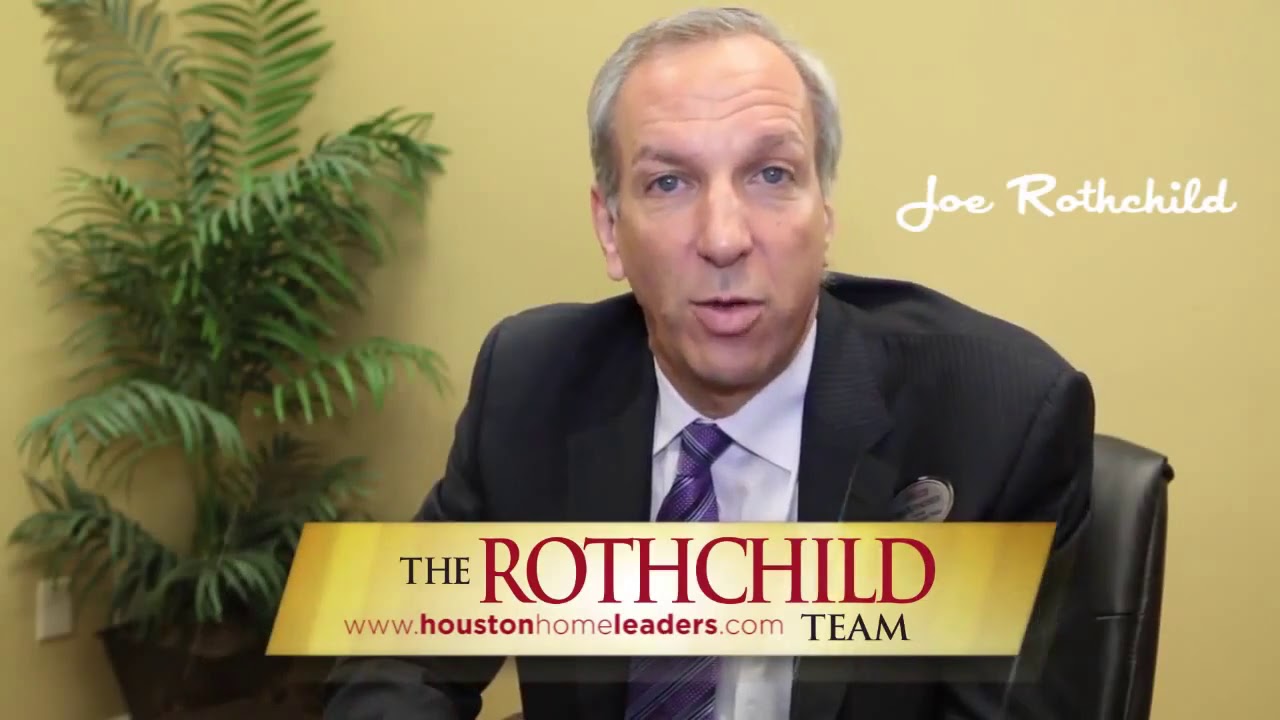In this advertisement image, we see an older gentleman named Joe Rothschild seated and centered. He has blue eyes, gray hair, and a pale peach complexion. Joe is dressed in a dark suit jacket, which is black or possibly dark bluish-gray, paired with a white collared shirt and a purple and white striped tie. You can discern the black desk chair he is sitting on, noticeable just below his left shoulder on the right side of the image. 

The backdrop features a pale yellow wall with a philodendron plant in a black pot located in the far left quarter of the image, extending vertically. The text "Joe Rothschild" is elegantly written in cursive at the top right of the image in white lettering. Below, across Joe's chest, is a banner that reads "The Rothschild Team" with "The Rothschild" in uppercase red letters and the accompanying web address "www.HoustonHomeLeaders.com" in a combination of light red and red letters, emphasizing "team" in black. The overall style and composition suggest this is an advertisement for The Rothschild Team's real estate services.